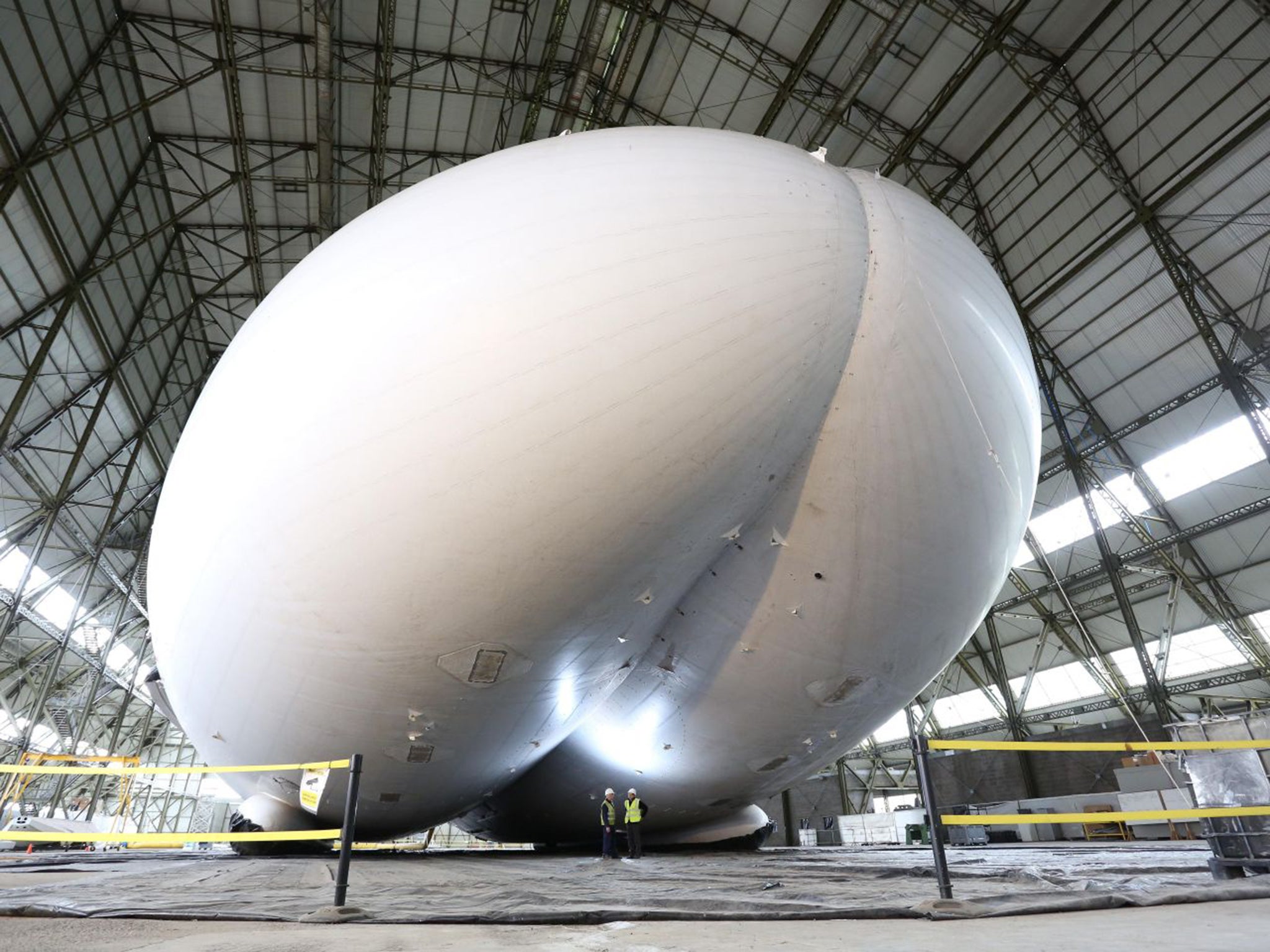In this detailed close-up photograph, we see a massive, white blimp dominating the frame, situated inside a colossal indoor facility. The blimp, which resembles two rocket ship-shaped objects fused together with an indent running vertically through its center, hovers impressively above the ground. Below, two small-scale workers in yellow safety vests, black long-sleeve shirts, white hard hats, and pants stand in conversation. Their hard hats are equipped with flashlights, reflecting light onto the blimp’s underside. The workers’ insignificance compared to the blimp highlights the sheer size of the enormous structure.

The blimp, with a somewhat translucent appearance, reveals streaks of gray under its white exterior, suggesting repairs with various patches visible on its surface. Its unusual shape, almost as if it has "legs and feet" but no top, adds intrigue. The facility itself, with its metal tower and numerous support beams, appears to provide a sheltered environment for the blimp. The area is somewhat open to the outside, evident from the visible barricades and the open section where people can enter. Lighting within the facility creates reflections on the blimp, giving the scene an industrial yet mystic ambience dominated by tones of gray, accentuating the blimp’s solid yet enigmatic presence.